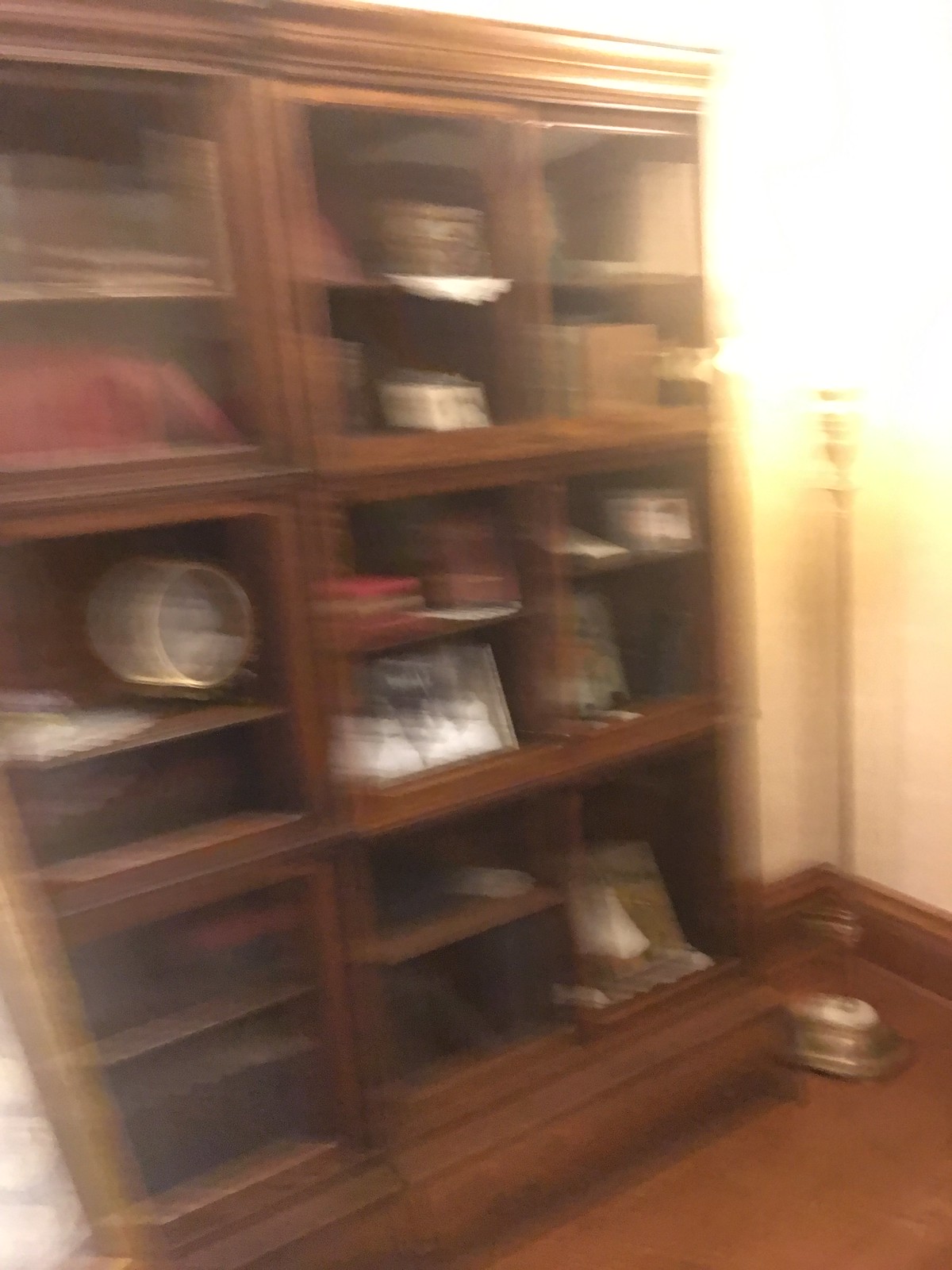The image is a somewhat blurry, color photograph of a dated, walnut-colored wooden breakfront, which is a piece of furniture with multiple shelves and compartments designed for display and storage. This large, vertical, rectangular cabinet is situated near the corner of a room with a brown wooden floor and white walls with brown baseboards. The breakfront features three main rows of shelves and compartments, with a variety of layouts across the rows. The top third and fourth rows have three compartments each, while the bottom section has two shelves on the left, two in the middle, and one open compartment on the end.

Inside the breakfront, there are various items including photographs, books, and a couple of canisters. Some compartments appear to have glass panes. Nearby, there's a tall, bright standing lamp with a metal pole, situated in the corner without a visible lampshade, casting a glare. The decor items and picture frames within the breakfront aren’t clearly visible due to the blurriness of the photograph.